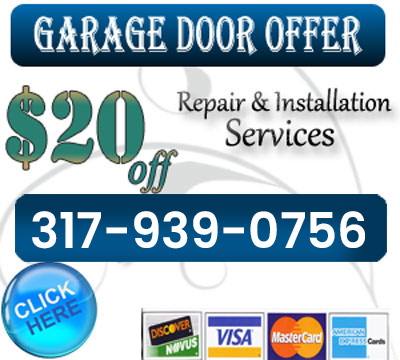This advertisement features a promotional offer for garage door services. The background is pristine white, accentuating a thin, subtle gray plant design that extends upward. At the top, a deep grayish-blue rectangle with rounded corners prominently displays the text "Garage Door Offer" in an elegant, sophisticated font. Below, on the left side, a green section highlights "$20 off," drawing attention immediately. On the right side, black text advertises "repair and installation services." At the bottom, bold text displays a contact phone number: 1-817-939-0756. Additionally, a clickable call-to-action button is situated at the bottom, designed like a bluish, glossy bubble that reads "Click Here." Various payment icons are also visible, suggesting multiple payment options are accepted.